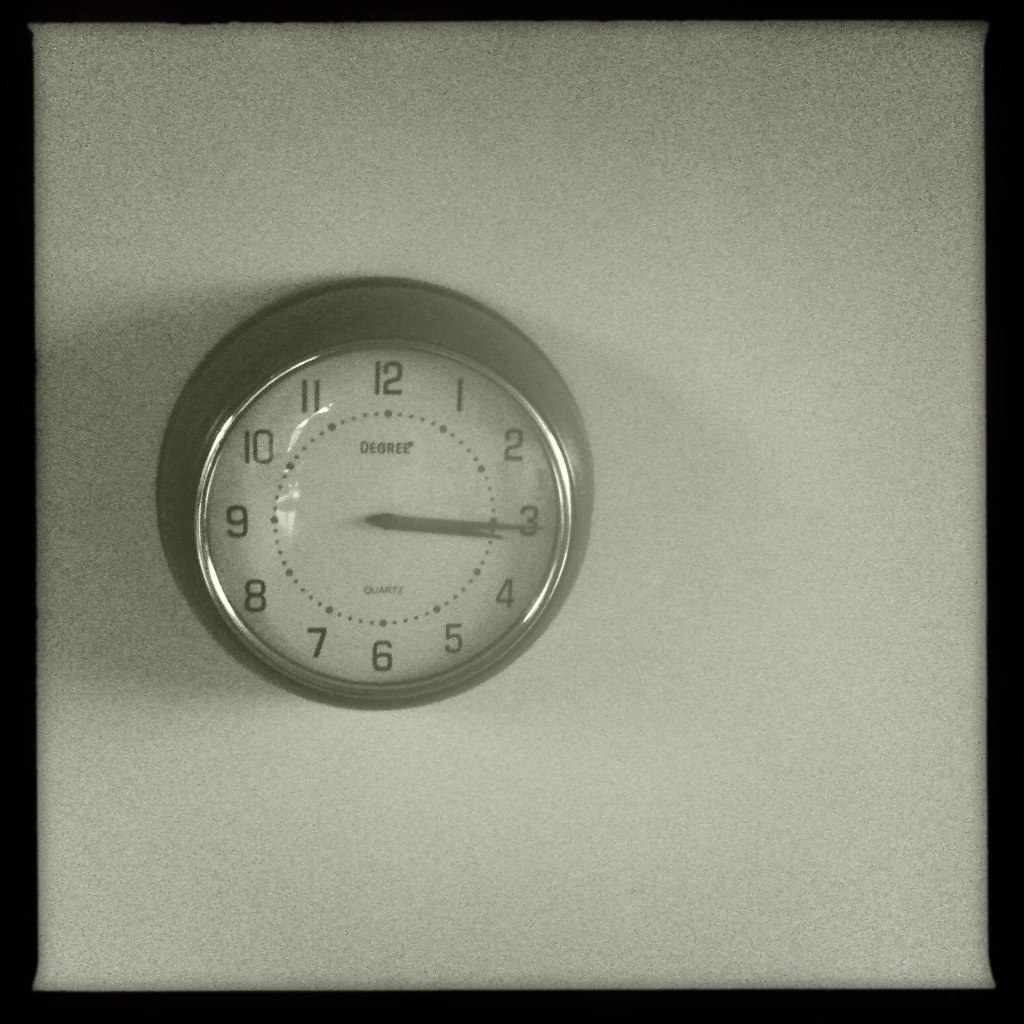A classic wall clock is mounted on a white, textured wall, reminiscent of those found in office buildings. Encased in a circular metal frame, the clock's face is stark white with bold black numbers. It features two black hands, indicating the time as 3:15 PM (close to 3:16 PM). The brand name "Degree" is inscribed near the center, while "Quartz" is noted at the bottom. Despite its simplicity, the clock serves as a functional timepiece with a traditional analogue design. The wall's subtle texture adds a layer of depth to the otherwise straightforward setting.